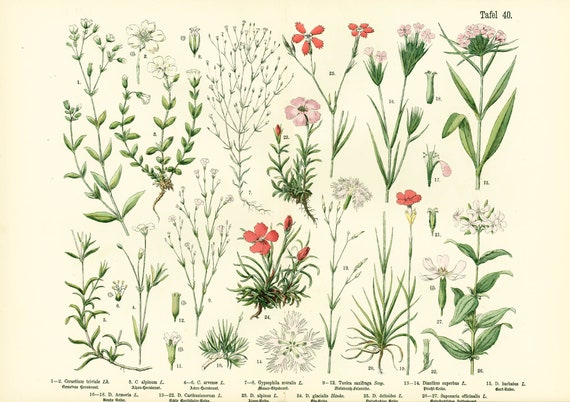The image depicts a detailed, possibly historical or scientific botanical illustration, showcasing a diverse collection of over 20 different types of flowers. The flowers are represented in a variety of colors including shades of red, pink, white, with occasional hints of yellow. The plants are illustrated with notable elements such as green stems, leaves, twigs, and grass. The flowers range in shape and form, with some featuring wide, robust petals while others have delicate clusters of tiny petals. Though there's text labeling each flower at the bottom, the font is too small to discern from the image provided. The top of the illustration is labeled "Tafel 40". This intricate diagram of flowers, reminiscent of something you might find in a library or museum, merges scientific accuracy with artistic detail, though it appears slightly aged or antiqued in nature.